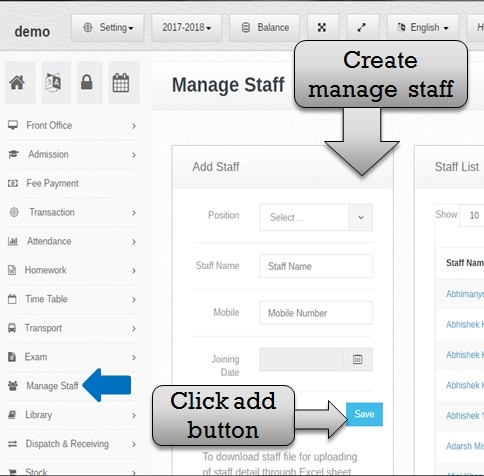The image is a detailed screenshot of a computer or mobile interface for a software application titled "Managed Staff." In the top left corner, the label "Demo" is prominently displayed, indicating a demonstration mode. The interface features a comprehensive side panel with various management options, including Front Office, Admission, Fee Payment, Transaction, Attendance, Homework, Timetable, Transport, Exam, Managed Staff, Library, Dispatch, and Receiving. 

Central to the interface is a section dedicated to managing staff, highlighted by a column titled "Add Staff" with a large arrow pointing down, directing the user to "Create Managed Staff." Additionally, there is another column labeled "Staff List" and below it "Staff Name," indicating fields that likely need to be filled out. 

Text bubbles guide users on how to navigate the interface, including a prominent gray bubble with an arrow and the text "Click Add Button." At the bottom of the screen is a significant and attention-grabbing blue button labeled "Save." 

The overall design is clean and well-spaced, with a color scheme consisting of gray, black, white, and shades of blue, ensuring readability and ease of use. This screenshot likely represents part of a web page or mobile application intended for streamlined staff management within an organizational setting.